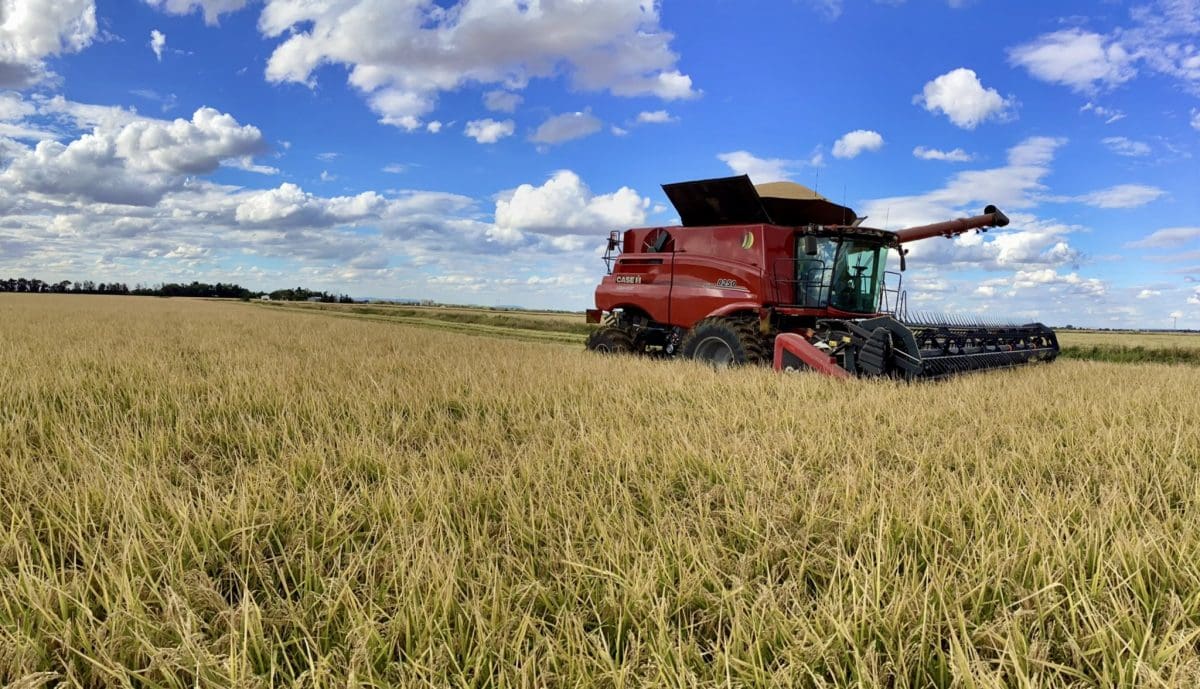The image features a large, shiny red combine tractor positioned centrally in a vast field of grain, likely wheat, oats, or barley. The tractor is equipped with a horizontal mower-style bar and red forks or arms at the front, which are used for cutting and collecting the grain. It has a clear cab for the driver and a grain chute or hopper on top. The tractor's large, black tires support its square build. The expansive fields stretching into the distance are green and golden, with a creamy hue to the tall grass heads. Far off in the background, there are trees and buildings, adding depth to the rural landscape. Overhead, the bright blue sky is dotted with fluffy white clouds, painting a picturesque daytime scene. Notably, there appears to be an emblem resembling a banana on the side or bed of the tractor.